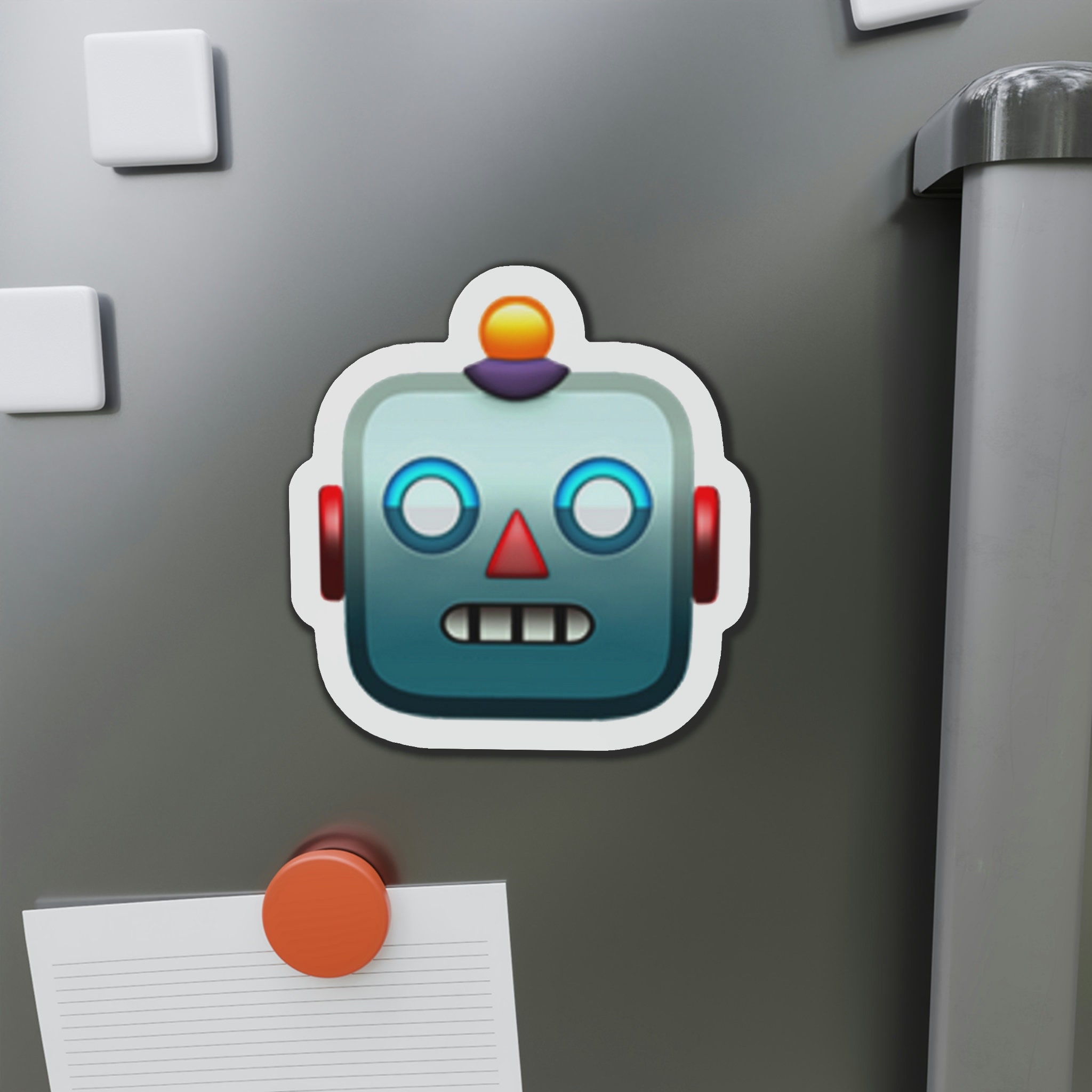This is a close-up image of a light gray refrigerator, featuring a central, vividly detailed magnet of a cartoonish robot emoji. The refrigerator's vertical handle is visible on the right side, highlighting a sleek, modern design. Surrounding the main magnet are several white square magnets, adding minimalistic accents to the fridge's surface. In the bottom left corner, a circular orange magnet holds a blank white postcard, creating a contrasting splash of color.

Dominating the scene, the robot magnet is a charming depiction with a grayish-blue face and blue eyes, outlined in teal. Its playful expression is accented with black lines for teeth, red triangle nose, and red circular ears. Topping off its head is a rounded receiver, featuring a yellow light and a purple mount, adding to its whimsical, non-threatening appearance. The magnet stands out not only for its size but also for its vibrant, friendly design, making it a fun and eye-catching decoration.